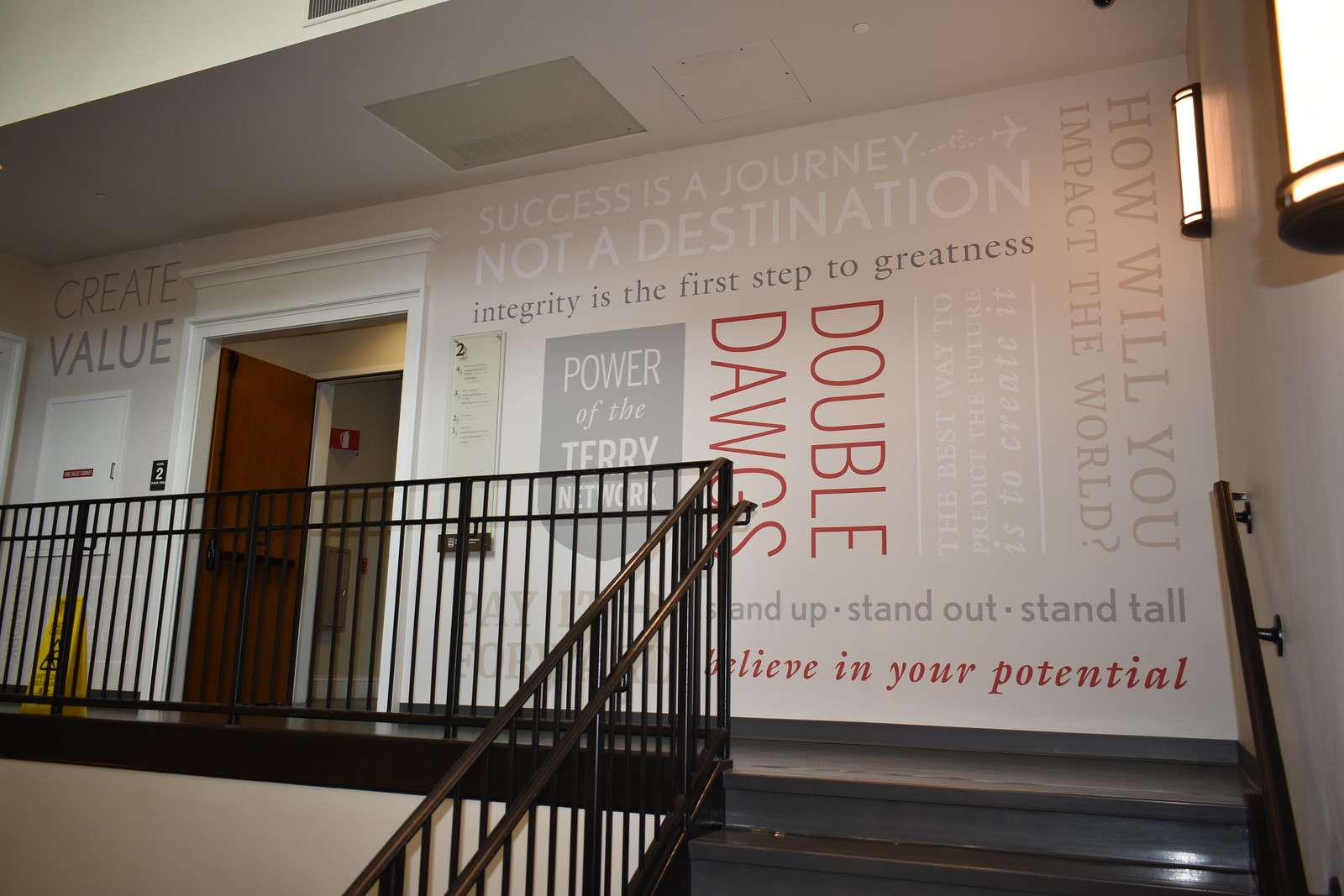Inside a building, the photograph captures a detailed interior view featuring a striking black staircase leading to a second floor. The staircase is equipped with a black handrail and is positioned at the bottom right corner, rising towards the center of the image. The wall on the second floor is painted white and adorned with a myriad of motivational quotes and phrases in various colors, sizes, and fonts.

Prominently displayed on this wall, you see, "Success is a journey, not a destination" in white letters next to a picture of a plane. Just below it, another quote reads, "Power of the Terry network" in a grey shield with white letters. Further along, the phrase "Double dogs" stands out in red letters, followed by "The best way to predict the future is to create it" in white letters, and "How will you impact the world?" in grey letters.

On the left side of the wall, there is another motivational message: "Create value" in grey letters, positioned above an electrical outlet box and near a yellow plastic "wet floor" caution sign. Directly next to this, there is a doorway with a white frame and a brown door. The overall color scheme of the interior includes white, grey, black, yellow, tan, and red.

Additional quotes scattered across the wall include, "Integrity is the first step to greatness" and below all other texts, "Stand up, stand out, stand tall, believe in your potential." The setting appears to be an indoor space, possibly a business or office environment.